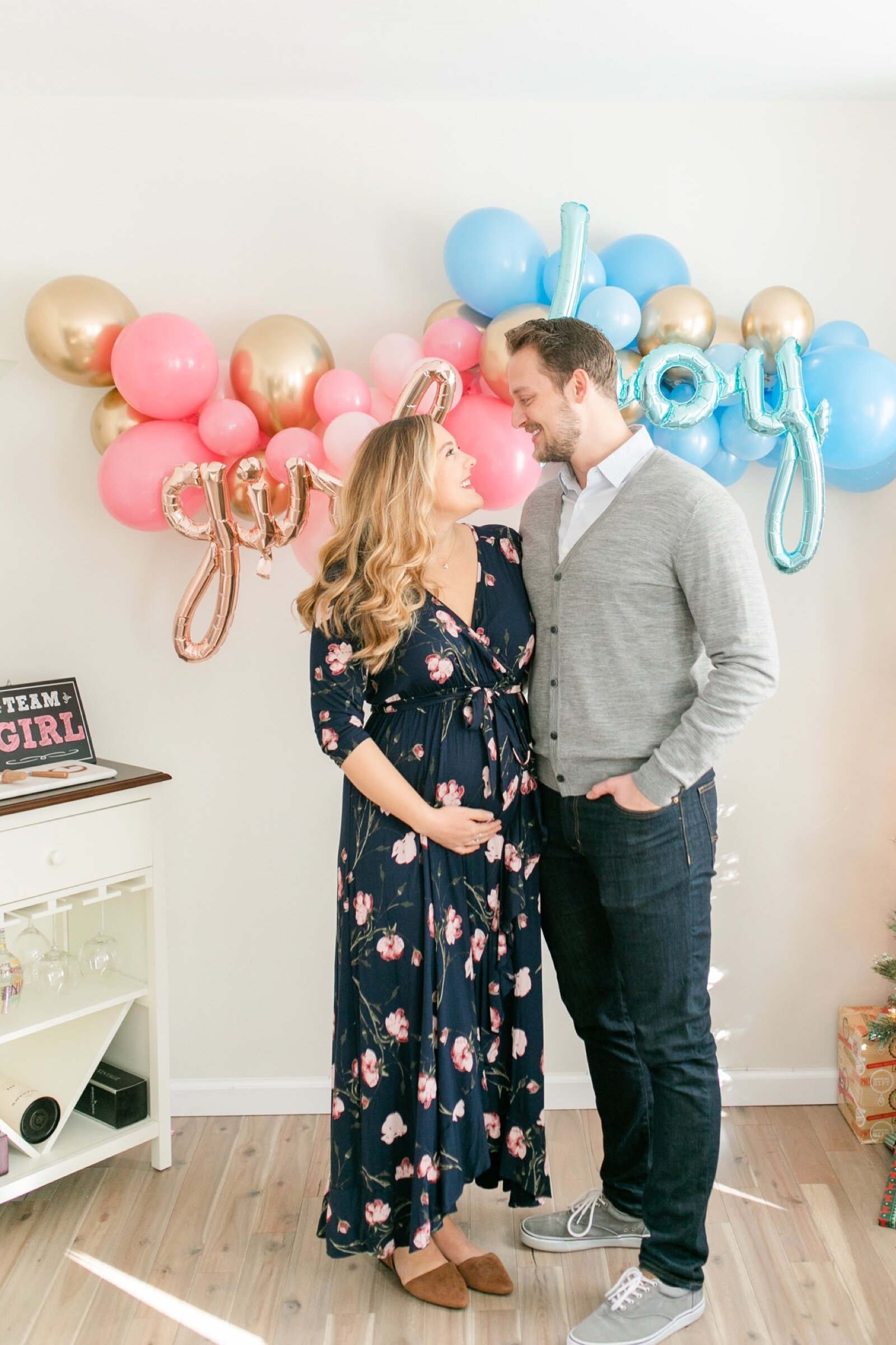In this detailed photograph of a gender reveal party, a central couple stands warmly embracing each other. The woman, positioned on the left, is visibly pregnant and exudes elegance in a navy wrap dress adorned with pink flowers. She has dark blonde hair and is wearing brown flat shoes, her arm lovingly wrapped around the man beside her. The man, slightly taller, sports a scruffy beard and is casually dressed in a light gray cardigan sweater over a white shirt, paired with blue jeans and gray canvas shoes. Both are gazing affectionately at each other, encapsulating the joy of the moment.

Behind them is a festive balloon display, divided into two sections. On the left, pink and gold balloons cluster around a large balloon that declares "girl," while on the right, blue and gold balloons frame a balloon that reads "boy." Further emphasizing the theme, a sign that reads "team girl" is perched atop a white wine cabinet with a brown top to the left of the couple, suggesting a strong leaning towards one gender. The scene is set on a light hardwood floor, with a very pale beige wall in the background, contributing to the photo's warm and inviting ambiance. Additionally, on the right side of the image, there are glimpses of what appear to be wrapped gifts and a table or box, adding to the celebratory atmosphere.